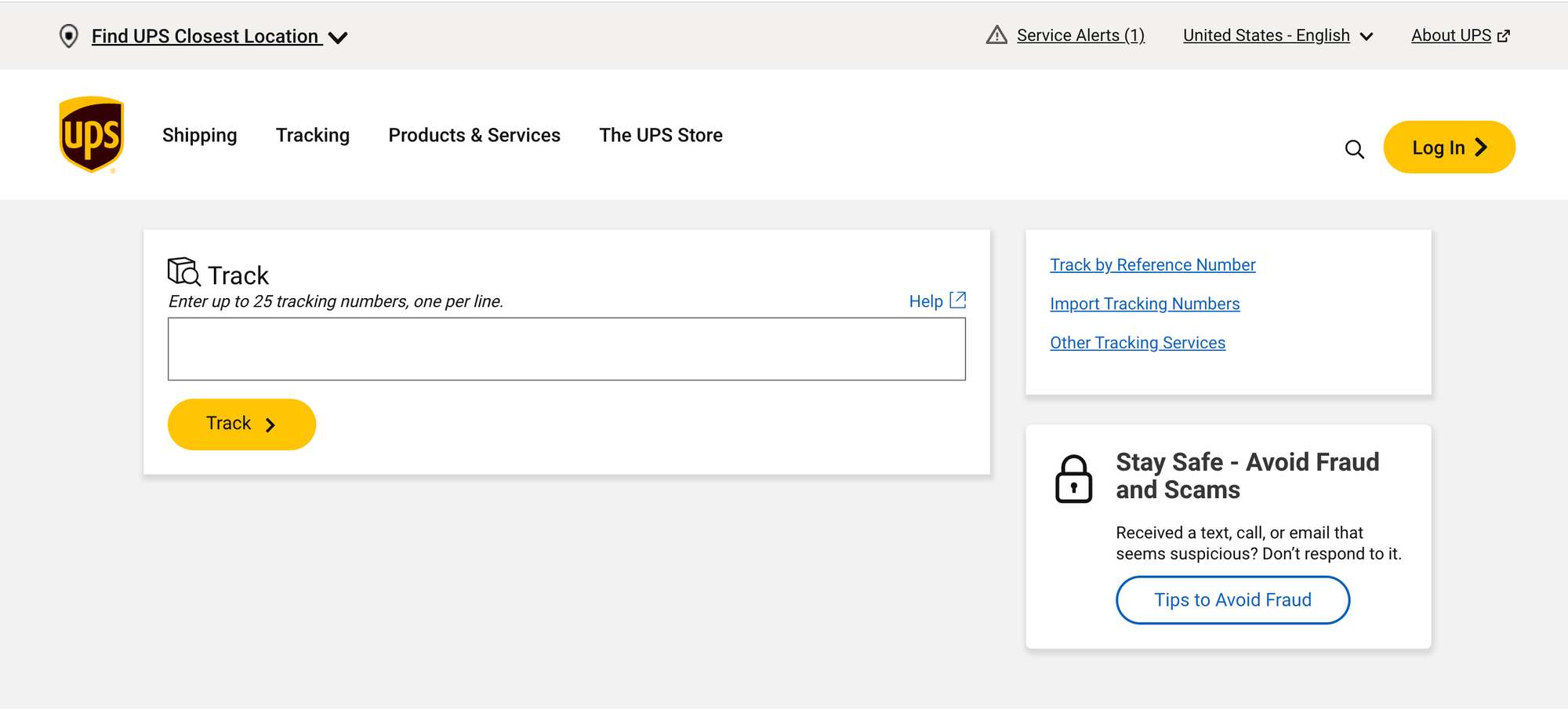The screenshot captures a webpage dedicated to locating the nearest UPS location. The top of the page features a gray border with a pin drop icon labeled "Find UPS Closest Location" accompanied by a drop-down arrow. To the right are buttons for "Service Alerts," "United States" with an English language drop-down, and "About UPS".

Below this is a white border with the UPS logo positioned in the upper left corner. The logo features a shield design, with a yellow top portion and a black main section, displaying "UPS" in yellow letters. To the right of the logo are navigational tabs: "Shipping," "Tracking," "Products and Services," and "The UPS Store". On the far right, there is a search icon followed by a yellow login button.

The primary interface has a gray background with a prominent white rectangle in the center labeled "Track". Within this rectangle, the text instructs users to "Enter up to 25 tracking numbers, one per line," and features an input box beneath this instruction. Below the input box, a yellow button labeled "Track" is visible.

To the right of this central section are two additional rectangles. The top rectangle is divided into three blue-tinted sections titled "Track by Reference Number," "Import Tracking Numbers," and "Other Tracking Services." The bottom rectangle includes a black padlock icon accompanied by the text "Stay Safe, Avoid Fraud and Scams." It advises users to ignore suspicious texts, calls, or emails, and features a blue oval button labeled "Tips to Avoid Fraud".